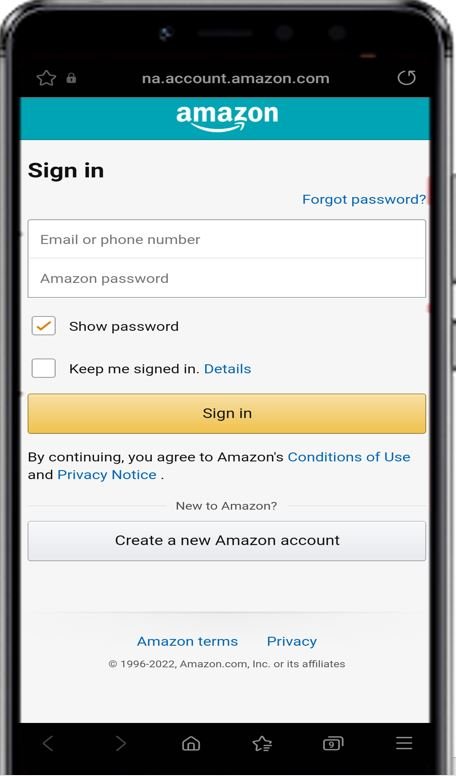The image showcases a smartphone in portrait orientation, positioned against a stark white background with no defining borders. The cellphone features a black frame with a glossy gray outer material and rounded edges, making it distinctly taller than it is wide. At the top of the phone's display is a horizontal search bar with elements including a hollow star icon (for favorites), a lock icon, and the text 'na.account.amazon.com' followed by a refresh button.

Beneath this, the screen prominently displays a blue horizontal bar with 'Amazon' written in white font. Below this bar is a gray section featuring 'Sign-In' in black lettering to the upper left and 'Forgot Password' to the upper right. Further down, there are two white input fields labeled 'Email or mobile phone number' and 'Amazon password' respectively.

Directly underneath these input fields, there are two options regarding password visibility and session retention: a checked box next to 'Show password' and an unchecked box next to 'Keep me signed in.' Below these, a horizontal yellow button with 'Sign-In' written in black font beckons the user to proceed.

At the bottom of the screen, a notice in black font reads, "By continuing, you agree to Amazon's Conditions of Use and Privacy Notice," accompanied by a link to create a new Amazon account if necessary.